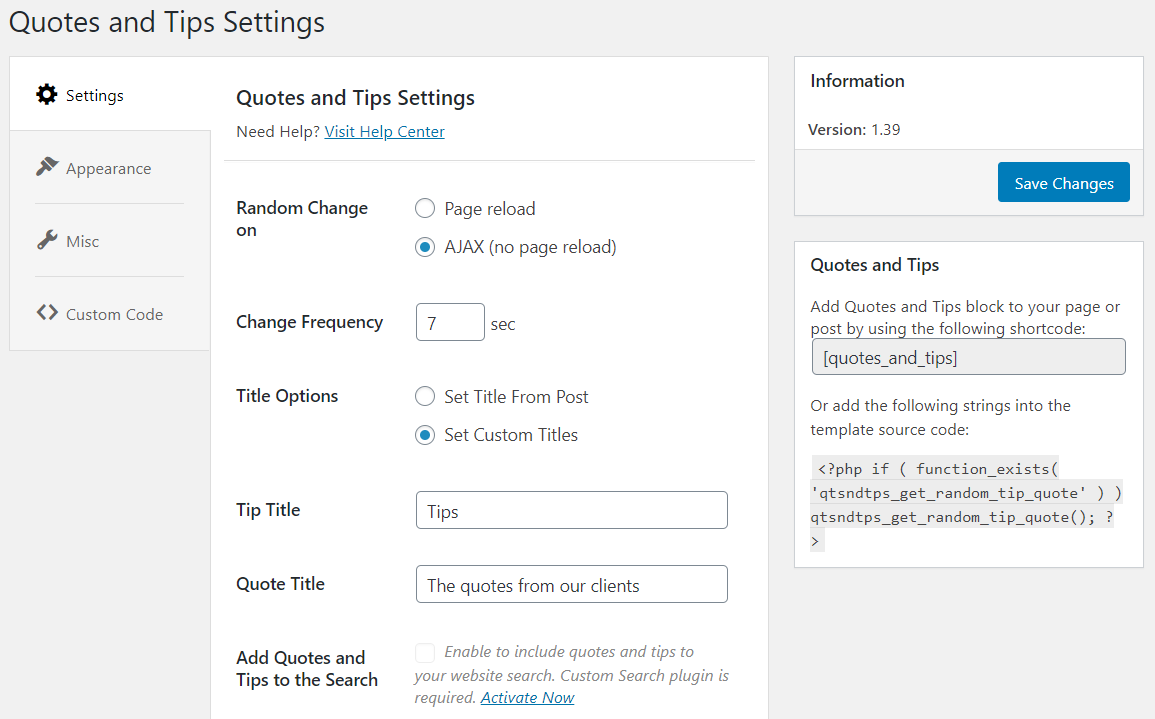This image displays a screenshot of an application interface, although the specific platform is indeterminate because the surrounding UI elements are not visible due to the cropping of the screenshot. The interface features an off-white grayish background with distinct sections that draw the viewer's attention using a white backdrop. Blue is utilized as an accent color for selected items and buttons, including a "Save Changes" button located on the right side. There are also several blue hyperlinks scattered throughout the interface.

At the top, the main title reads "Quotes and Tips Settings," immediately followed by a vertically arranged, tab-style menu. The menu's top item, "Settings," is currently selected, and is denoted by a gear icon. Other menu items include "Appearance," marked with a brush icon, and grayed-out options: "Miscellaneous" with a wrench icon, and "Custom Code" with two brackets.

Beneath the section header "Quotes and Tips Settings," the white background area highlights multiple configurable options. These options feature black text and include:

1. "Random Change On" with a radio button.
2. "Change Frequency," likely accompanied by a text input field.
3. "Title Options," encompassing various sub-options like "Tip Title" and "Quote Title."
4. "Add Quotes and Tips to the Search" with associated descriptions.

On the right side of the screen, a section titled "Quotes and Tips" provides instructions for adding these elements to a page or post using shortcodes. This section includes a copyable box with one shortcode and an alternative option listed below it, consisting of three lines of template shortcode.

The overall design of the application is clean and organized, leveraging color contrasts and iconography to guide users through their configuration options efficiently.